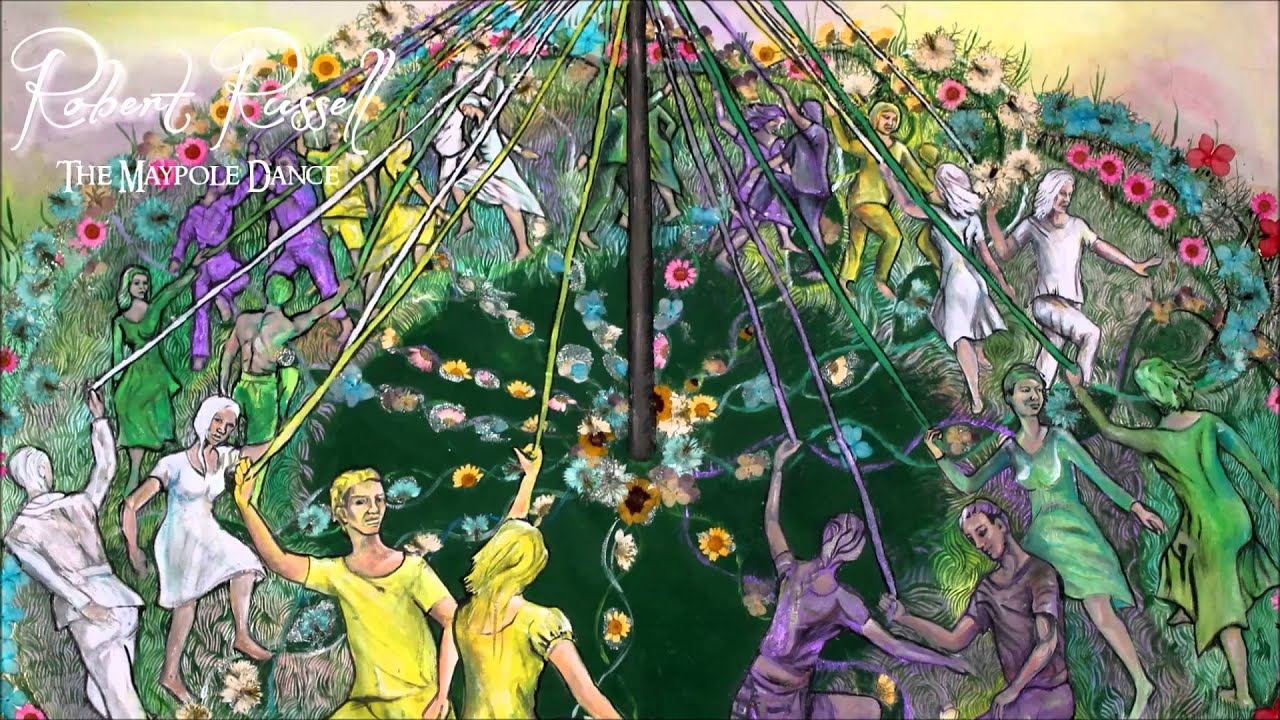This vibrant painting by Robert Russell, titled "The Maypole Dance," captures an array of multicolored figures dancing around a central maypole. The pole, painted in dark brown with pink accents, stands prominently in the center of the composition, adorned with cascading flowers at its base that spiral outward. Each dancer, depicted in striking hues of yellow, purple, green, and white, holds a ribbon extending from the pole, forming a lively circular formation on lush grass. The dancers' clothing and hair match their vibrant colors, adding to the surreal and almost psychedelic atmosphere of the scene. The sky above gradients through various shades of pink, further enhancing the dreamy quality of the artwork. Delicate flowers in a spectrum of colors, including orange, yellow, light blue, and purple, add to the intricate details surrounding the dancers. The painting is signed in the upper left corner by the artist, Robert Russell, accompanied by the title "The Maypole Dance," presented in a white script.